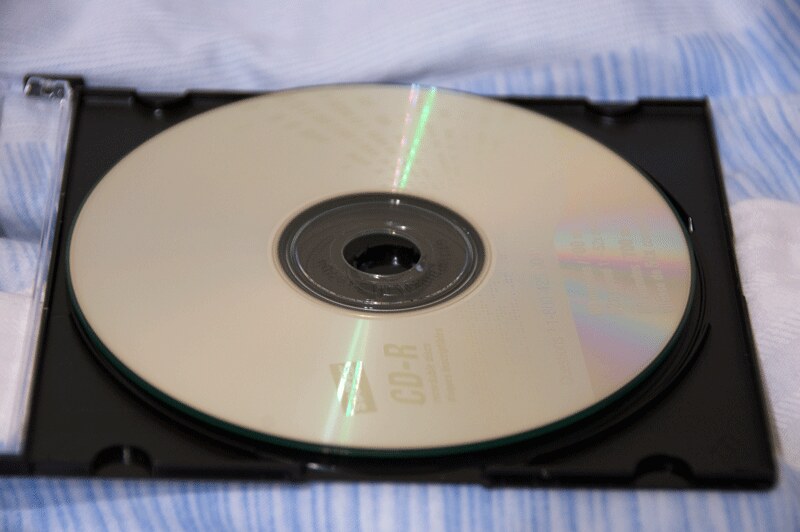The photograph, taken indoors, depicts a CD-R in its open, clear case with a black backing, lying on a piece of cloth. The cloth, resembling a bedspread or comforter, is predominantly white with numerous tiny blue lines. The CD itself is a blank, silver-to-gold colored disc, typically used for burning personal music. Printed on the CD is "CD-R". The disc appears slightly detached from the part of the case that usually holds it securely.